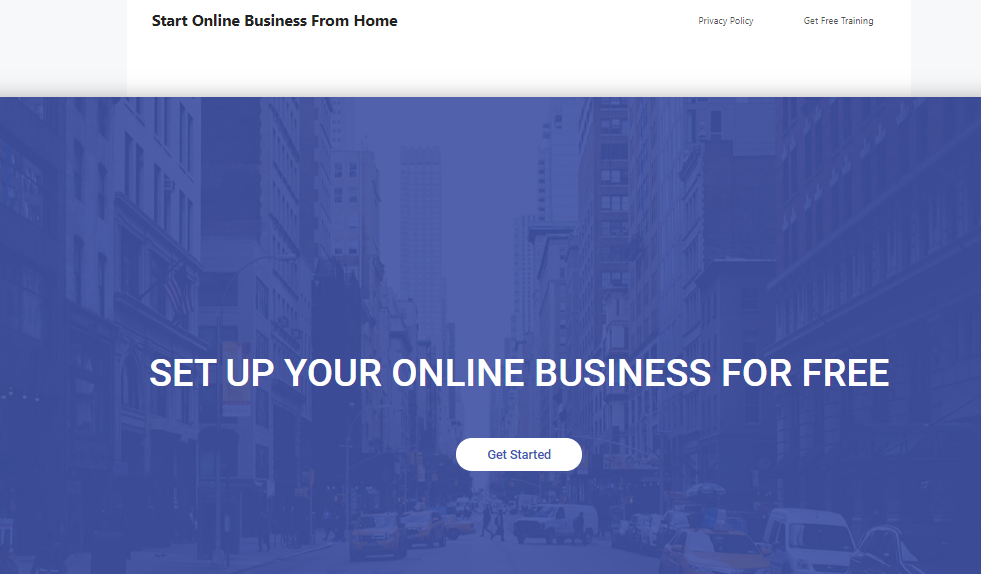This image depicts a promotional webpage for setting up an online business from home. At the top left corner, the header "Start Online Business From Home" is displayed in black text next to a small light gray box. The top right corner features links to "Get Free Training" and the "Privacy Policy," with another light gray rectangular box nearby. Dominating the center of the page, the message "Set up your own online business for free" is prominently showcased, accompanied by a rounded rectangular button labeled "Get Started" beneath it.

The background reveals a cityscape with a bluish tint, illustrating an urban environment. At the bottom middle, a straight road flanked by cars, including two yellow taxis on the left, can be seen. Two pedestrians are actively crossing the street, bringing life to the scene. An American flag is visible towards the middle left, adding a touch of national identity. Above, the sky is clear and free of clouds, completing the backdrop with a serene atmosphere.